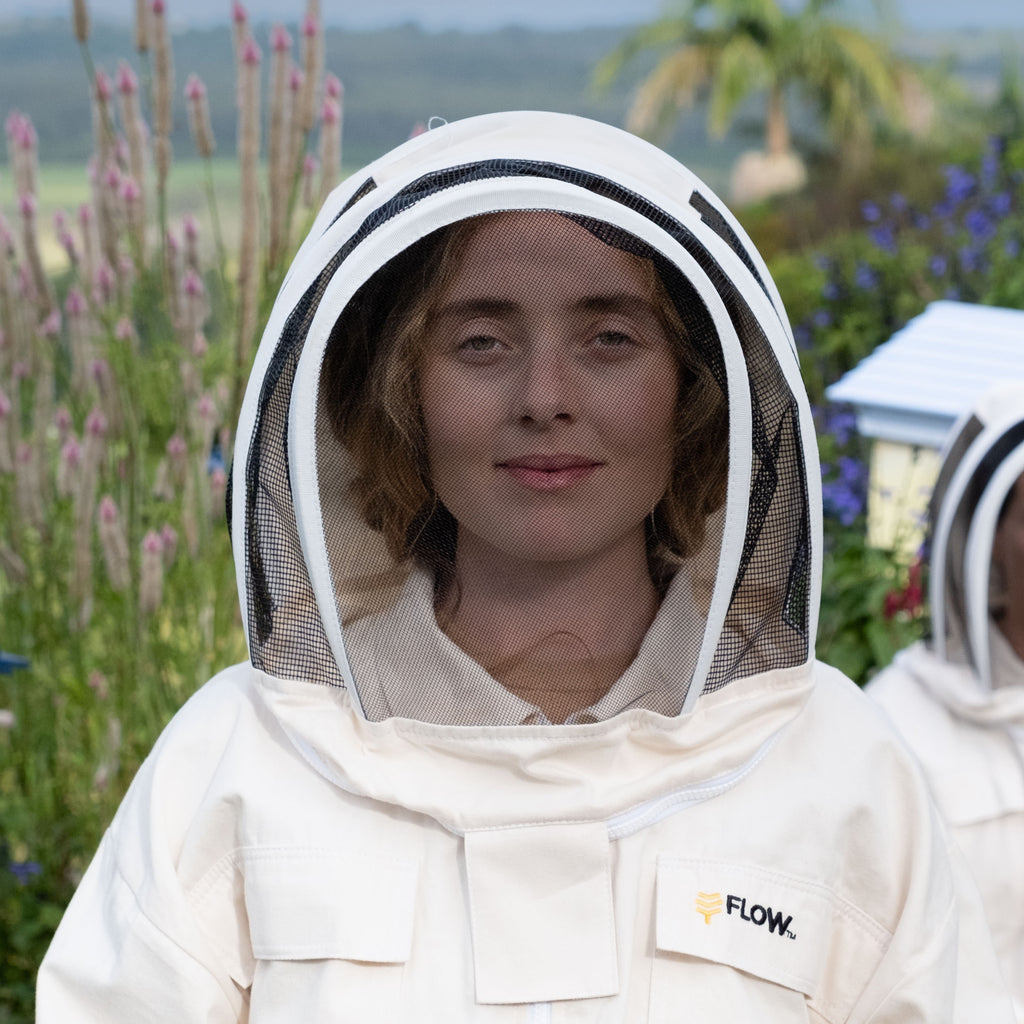The photograph is a full-color, vertical rectangle featuring a young white woman, aged 20 to 25, smiling warmly in the center. She is dressed in a white beekeeper's outfit, complete with a black mesh screened hood over her head and the word "FLOW" written on one of the lapels. Her short brown hair is visible beneath the netting. To her right, a second person, similarly attired, is partially visible with only a small part of their body and face showing. Behind her, there is a blend of tall vegetation and flowers, alongside a yellow and white building that resembles a small shed or wooden structure. On the left side of the image, a field of flowers stretches out, adding to the vibrant, natural setting. The background also includes some blurred greenery and what appears to be a pond, providing a great depth of field while keeping the smiling woman in sharp focus.